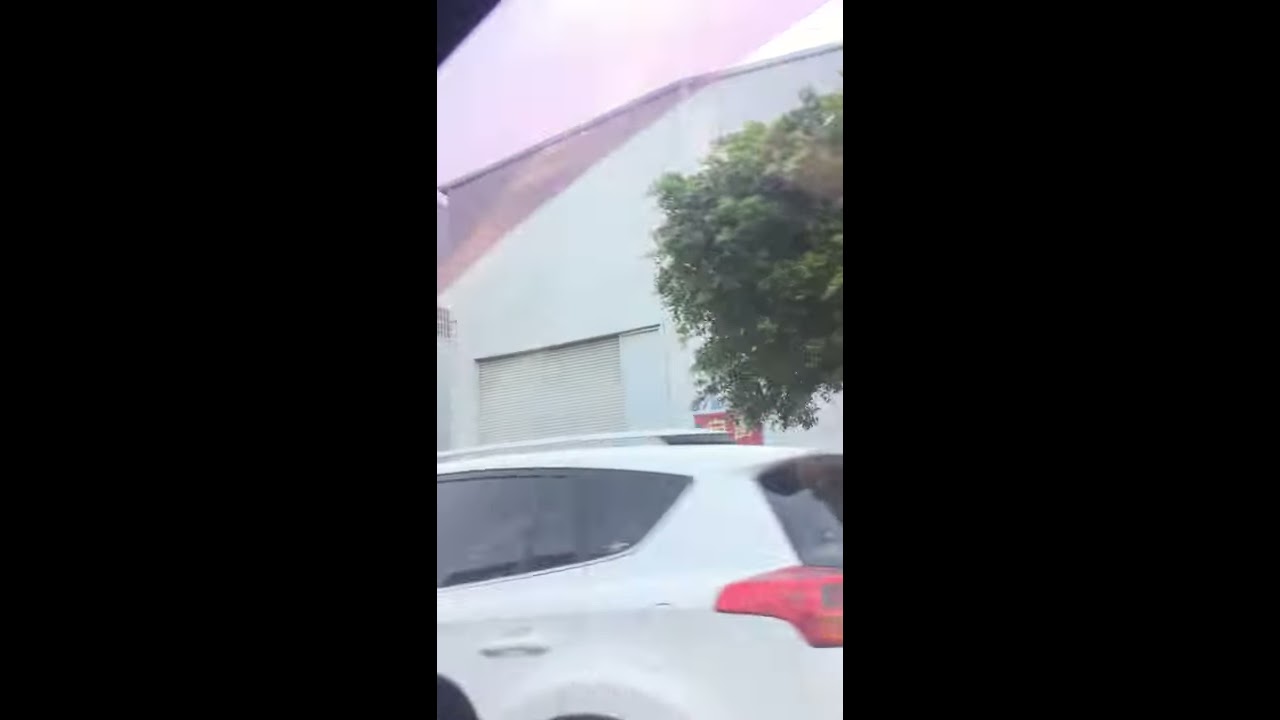The low-quality, horizontal image appears to have been taken through the window of another moving car, creating a sense of motion. At the bottom half of the image, a white car, likely a hatchback or SUV, is prominently featured, though only the rear part with dark windows is visible. The wheels and door handles are barely discernible. The car looks parked under the foliage of a green tree, part of which is visible on the right side of the frame. In the background stands a large, warehouse-like building painted a very light blue with purplish accents near the roof. The roof area of the warehouse is painted a lavender color with a white edge, and there's what appears to be a garage door. A red item, possibly a shopping cart, is parked in front of the building. The scene is set outside on a bright, mid-day, with the sun casting ample light on the surroundings. The image is framed vertically within a horizontal screenshot, leaving black borders around the main scene.